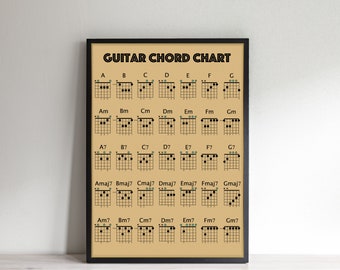This photo features a framed poster of a guitar chord chart, leaning against a white wall. The simple, thin black frame—likely made of wood—encases a kraft paper-colored poster with bold black ink. Prominently, the top of the poster is labeled "Guitar Chord Chart" in large, black lettering. The chart itself methodically lists various chords, starting with the most common chords from A to G on the first row. The second row contains minor chords, while the third row displays fifth and seventh chords (e.g., A7, B7, C7, etc.). The fourth and bottom rows presumably show major and major seventh chords. Each chord name is accompanied by a detailed fretboard diagram indicating finger placements on the strings. Natural light casts a soft shadow of the poster to the right on the white wall, adding depth to the image.